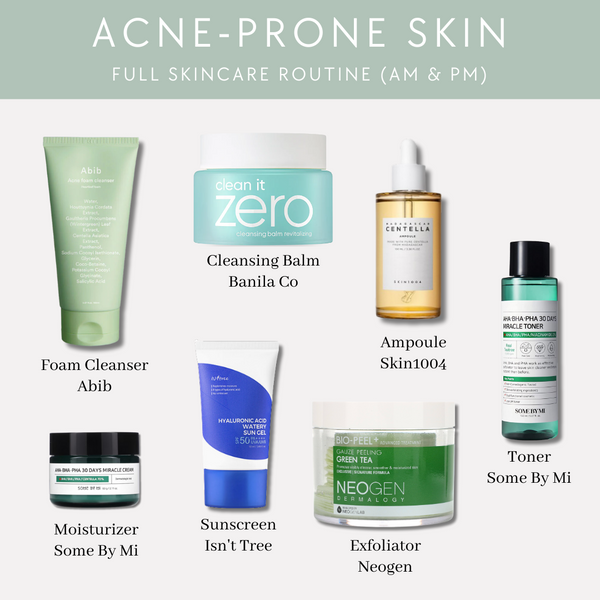This advertisement showcases a comprehensive skincare routine specifically designed for acne-prone skin, suitable for both AM and PM use. The top features a sage green horizontal banner with large white letters stating "Acne-Prone Skin" and "Full Skincare Routine (AM and PM)" prominently in the center. The background is a very light gray, creating a clean and minimalist aesthetic.

At the bottom of the banner, a variety of beauty products are displayed with their names listed beneath them in black font. From left to right, the products include:

1. **Foam Cleanser** by Abib, packaged in a light green tube with white writing.
2. **Cleansing Balm** by Nila Co, housed in a light sky blue jar with a white lid, labeled "Clean it Zero" at the top.
3. **Ampoule** by Skin 1004.
4. **Toner** by Somme by me.
5. **Exfoliator** by Neogen.
6. **Sunscreen** by Isntree.
7. **Moisturizer** also by Somme by me.

These products form a complete regimen aimed at smoothing and improving the condition of acne-prone skin, making it less susceptible to breakouts. The clean, orderly display and detailed product descriptions convey the effectiveness and targeted nature of the skincare solutions offered.